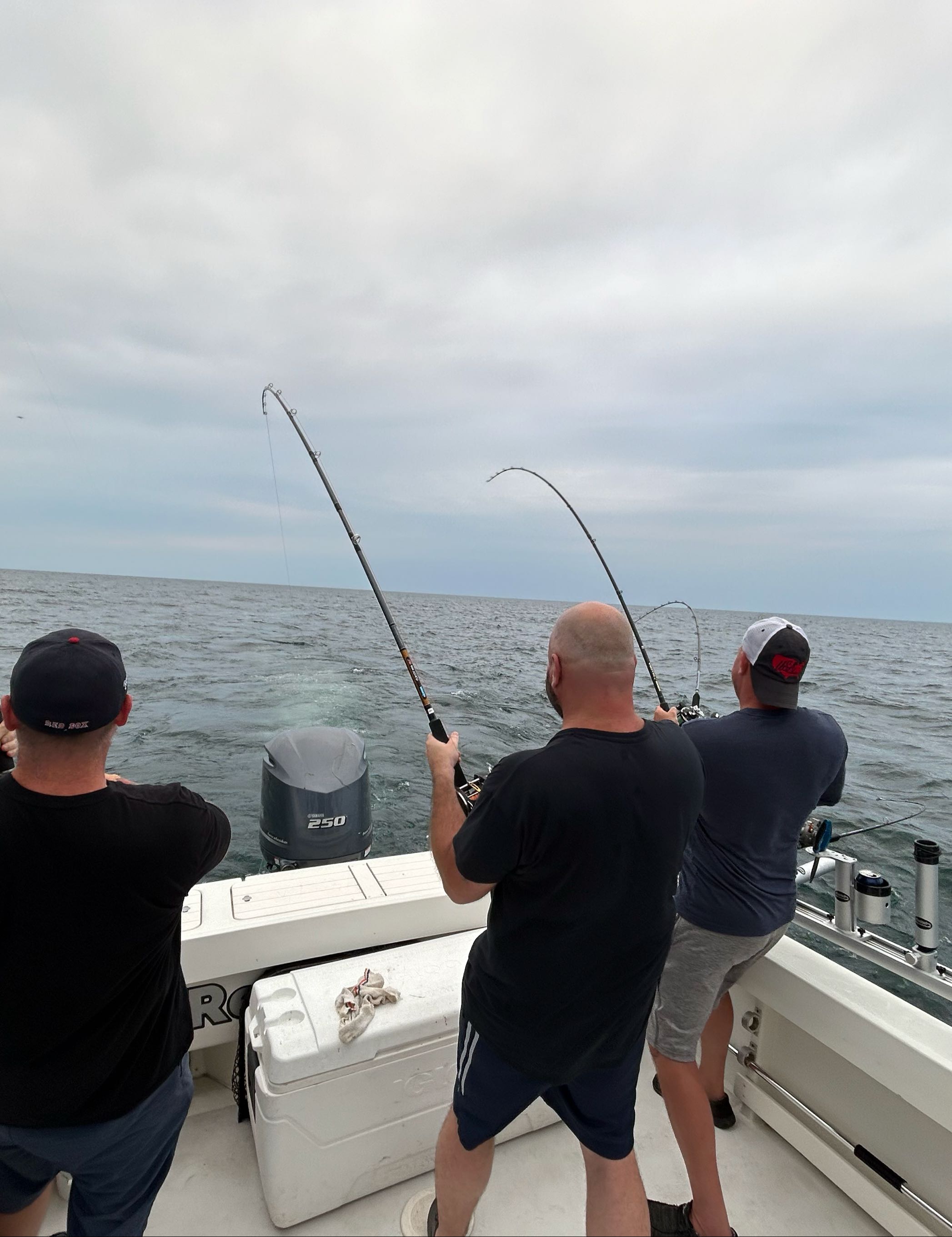In this image, three men are fishing off the back of a white-bottomed boat under a mostly gray, cloud-blanketed sky with hints of blue. All three men are wearing dark shirts. 

On the left, the first man is dressed in a black t-shirt, blue jeans, and a black hat, facing out towards the ocean. To his right, the second man is sporting a black shirt and black shorts, gripping a fishing rod that is notably bent, indicating a catch. Further to the right, the third man, wearing a blue shirt, gray shorts, and a backwards hat, is near two bent fishing rods, suggesting either multiple catches or rods attached to the boat. 

In front of the two men on the right, a cooler with a cloth or rag on top is situated. Additionally, there's a visible boat motor labeled "250" at the back. The clean, blue waters around them reflect the sky, and the atmosphere suggests that they are enjoying their time fishing together.